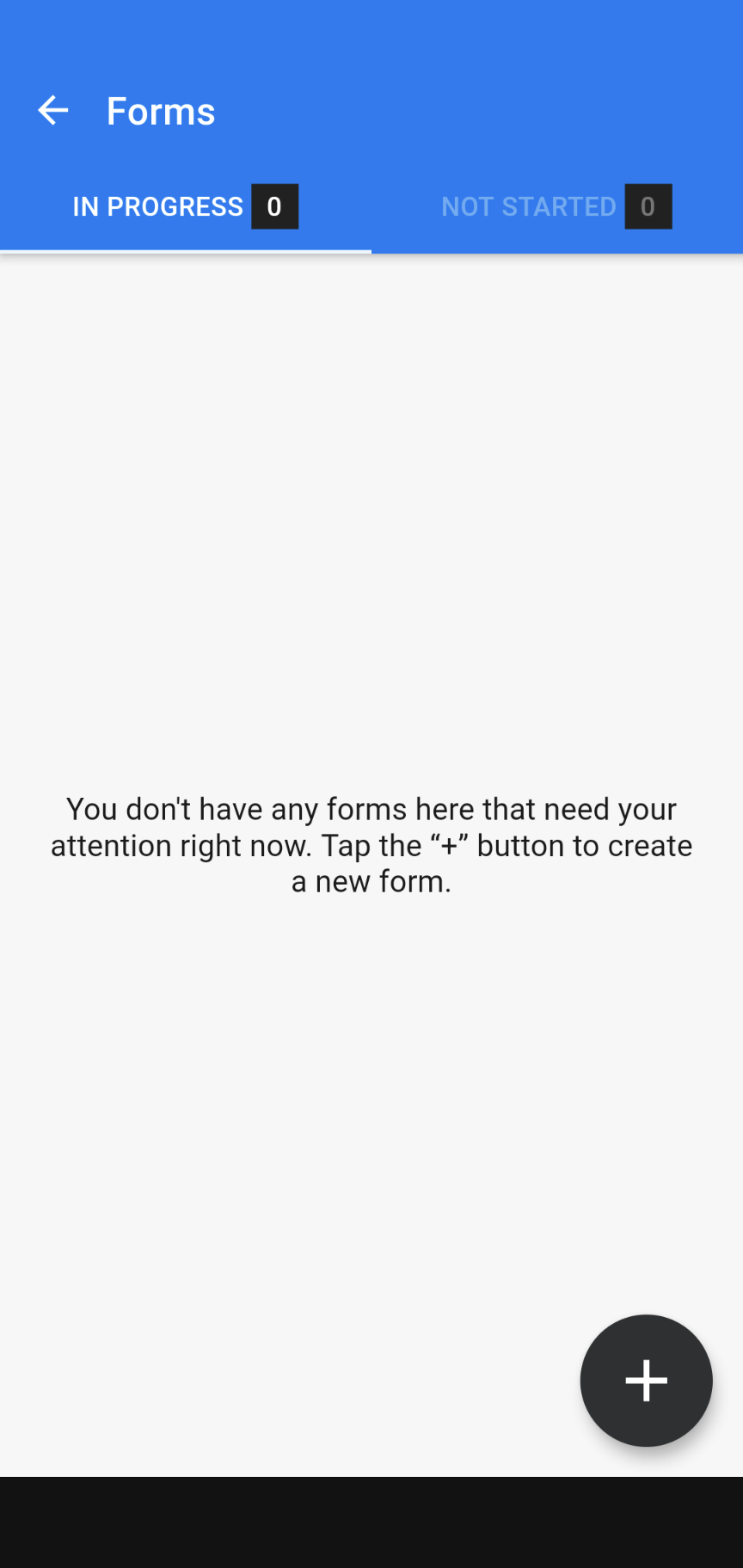This image, captured from a cell phone screen, displays a user interface within a form management application. The upper section of the screen is dominated by a royal blue background. At the top left, a white left-pointing arrow is accompanied by the text "Forms," also in white. 

Beneath this blue header, the middle section shifts to a faint gray background. Here, two status indicators are displayed: "In Progress" with a white zero encased in a black box, and "Not Started" with a zero next to it, both presented in black text against the gray background.

The lower section of the image features a solid black rectangular bar stretching horizontally across the screen. To the left within this bar, a black circle contains a prominent white plus (+) sign.

Spanning the middle section, centered in black text, is an instructional message: "You don't have any forms here that need your attention right now, tap the plus button to create a new form." This message is designed to guide users on creating new forms by using the plus button situated at the bottom left of the screen.